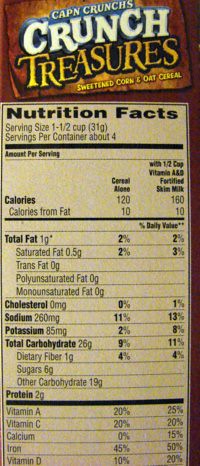The image is a photograph of the side of a cereal box labeled “Cap’n Crunch's Crunch Treasures.” At the top of the box, there’s a brown and orange background with the name “Captain Crunch's” in white letters outlined in blue. Beneath it, “Crunch” is also in white letters with a heavier blue outline, and “Treasures” is in yellow letters bordered by black. There is a line of text below "Treasures" that reads "Sweetened Corn and Oat Cereal."

Occupying most of the image is the Nutrition Facts panel, set against a faded yellowish-tan background with a black outline. The panel lists details in black text:  
- Serving Size: 1-1/2 cups
- Servings Per Container: about 4

It further provides nutritional information including:
- Calories and Calories from Fat
- Total Fat: 1g (2% daily value)
- Saturated Fat: 0.5g (3% daily value)
- Trans Fat: 0g
- Polyunsaturated Fat: 0g
- Monounsaturated Fat: 0g
- Cholesterol: 1mg (0% daily value)
- Sodium: 260mg (11% daily value)
- Potassium: 85mg (2% daily value)
- Total Carbohydrates: 26g (9% daily value)
- Dietary Fiber: 1g (4% daily value)
- Sugars: 0g
- Other Carbohydrates: 19g
- Protein: 2g

Additional vitamins and minerals are listed at the bottom, showing their daily value percentages:
- Vitamin A: 20%
- Vitamin C: 20%
- Calcium: 9%
- Iron: 48%
- Vitamin D: 10%

The photograph is low-quality and grainy but clear enough to read the text. The percentage values for daily recommendations are prominently listed on the right-hand side of the panel.